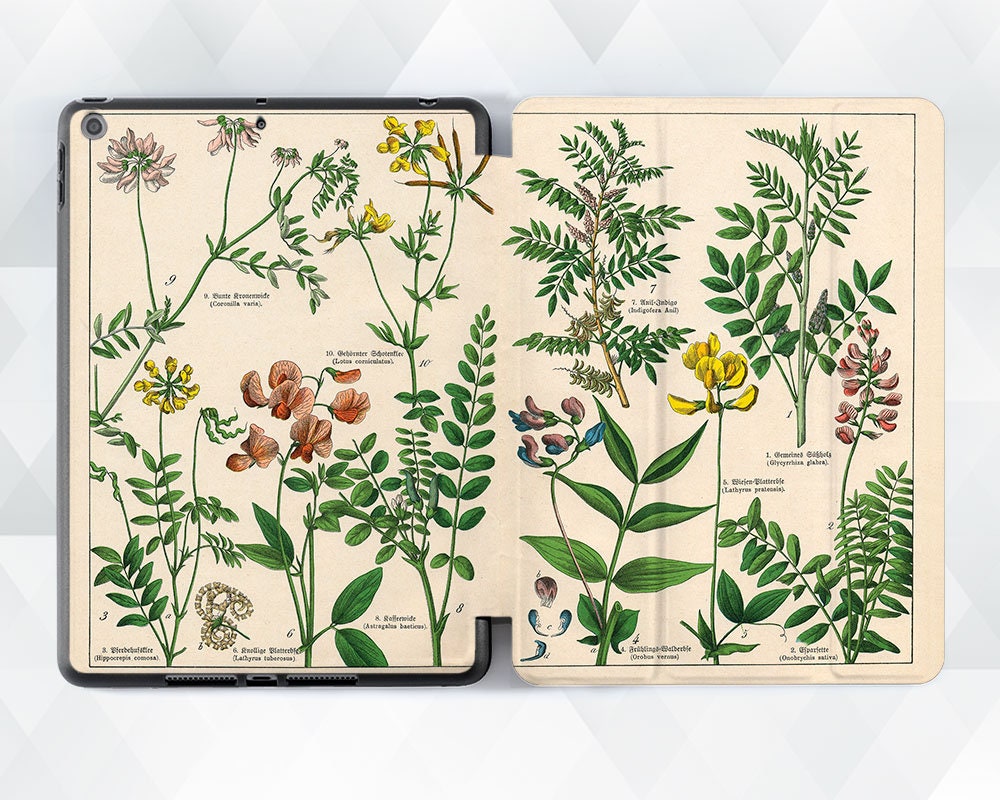This image is a detailed illustration showcasing various types of plants and flowers. It appears to be an info card or a diagram that features clean, full-color sketches of the plants, with vibrant green stems and leaves. Some plants are adorned with yellow, pink, or orange blossoms, while others are without flowers. Each plant is accompanied by text that identifies it, although the text is too small to read, likely containing long, scientific names. A notable detail is a light brown and white striped snake curled up among the leaves on the left side of the image. The rectangular illustration has an abstract, acrylic-colored background with some triangular shapes and is framed by an odd structure on the left that is not easily identifiable. The images are centrally positioned, dominating the space and drawing the viewer's focus.